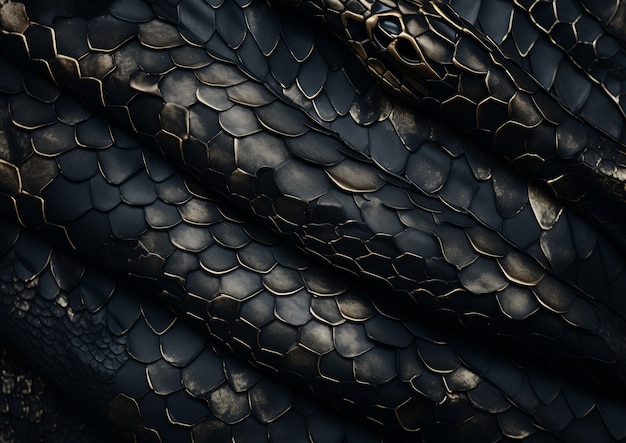This highly detailed and textured image appears to depict a computer-generated representation of a snake's body, focusing on its scales. The snake's body is wound in a complex, overlapping pattern, creating a series of cylindrical, tube-like shapes without showing the head. The scales exhibit a metallic sheen with a color palette dominated by dark hues, ranging from deep blue and black to brown and gray. Highlights of gold and silver add a luminous quality to some of the scales, enhancing their three-dimensional appearance. The scales are primarily hexagonal or octagonal and vary in color with some displaying white and highlighted edges, creating a visually intricate and abstract effect reminiscent of modern art. The diagonal ridges formed by the overlapping scale pattern extend from the bottom right to the top left of the image, emphasizing the snake's coiled form. There are no other objects or text present in the image, making the scales' detailed texture the focal point.